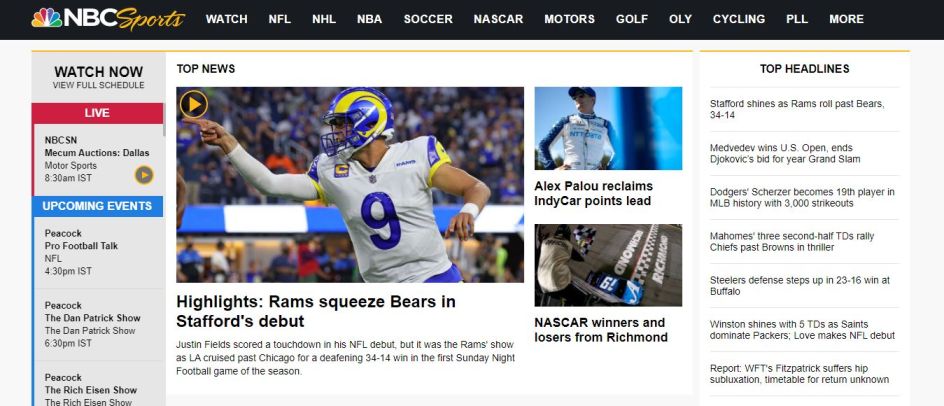This image is a screenshot taken from the NBC Sports online page. The background is predominantly black, providing a sleek, professional look. At the center of the image, there's the iconic NBA logo, which is artistically designed to resemble rainbow feathers encircling a white intersection.

At the top, the background remains black, overlaid with white text listing various sports categories in a rectangular segment. The categories include: "Watch NFL, NHL, NBA, Soccer, NASCAR, Motors, Golf, Ollie, Cycling, PLL, More." Just below these categories, there are options on either side to "Watch Now" or "View Full Schedule."

The page is divided into several sections, including one for live and upcoming events. Below these sections, there are a series of articles with highlights such as:

- "Rams Squeeze Bears in Stafford's Debut"
- "Alex Palou Reclaims IndyCar Points Lead"
- "NASCAR Winners and Losers from Richmond"

Additionally, there’s a sidebar on the right dedicated to "Top Headlines," featuring clickable links to several articles.

The NBC logo in the image features the letters "NBC" in white, accompanied by the word "Sports" in cursive, which is rendered in bright yellow, adding a touch of vibrancy to the overall dark-toned theme.